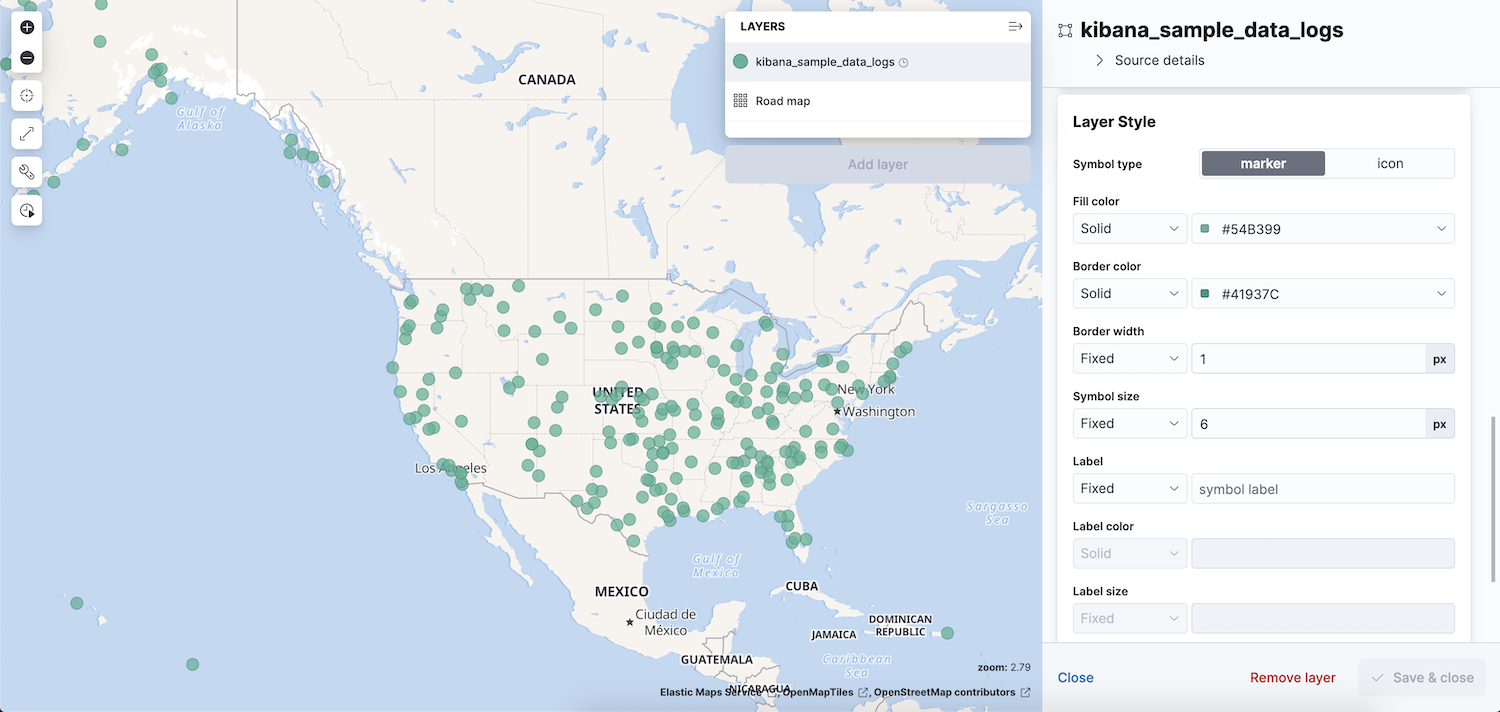In the screenshot, there is a Kibana interface prominently displayed. On the right-hand side, a filter panel titled "Kibana Sample Data Logs" is visible. Below this panel, there is a section labeled "Layer Style," which offers customization options such as Marker type (instead of Icon), Color, Border Color, Border Width, Symbol Size, Label, Label Color, and Label Size. At the bottom of this section, options for "Close," "Remove Layer," and "Save and Close" are displayed, with "Remove Layer" highlighted in red.

The central part of the screen features a map of the United States, displaying the geographical distribution of searches. The map extends to include neighboring countries like Mexico, Guatemala, Cuba, Jamaica, the Dominican Republic, and Canada. It is evident that the majority of search data points are concentrated in the United States, with several points appearing in western Canada. There is only one search point visible in the Dominican Republic, and no search points appear in the other mentioned areas.